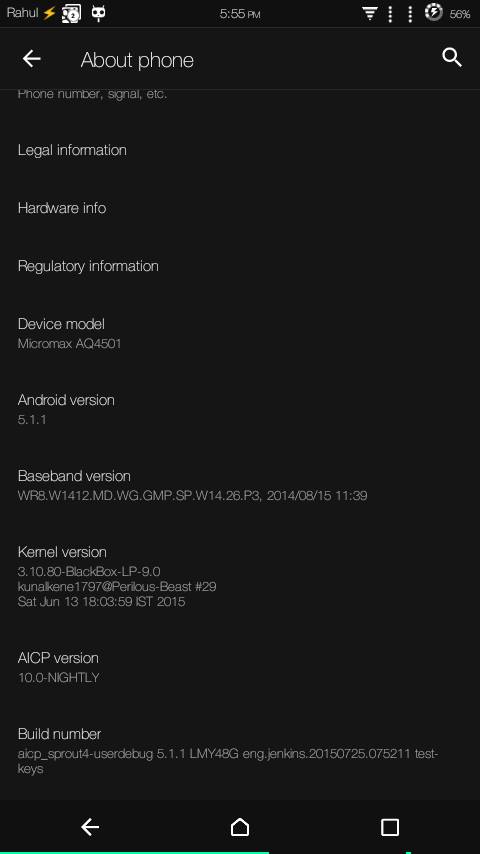This image captures the "About Phone" section of a mobile device, set against a black background. At the top, "About Phone" text is prominently displayed alongside a back arrow on the left, and a search icon on the right. Below this header, a section lists key details about the phone such as "Phone Number," "Signal," and other essentials. 

Further down, the list continues with categories like "Legal Information," "Hardware Info," and "Regulatory Information." The device model is specified as "Micromax AQ4501," followed by the "Android Version" details, which indicate version 5.1.1. The subsequent entries include the "Baseband Version," the "Kernel Version," and the "AICP Version," noted as 10.0-nightly. Concluding this detailed overview is the "Build Number" information provided underneath.